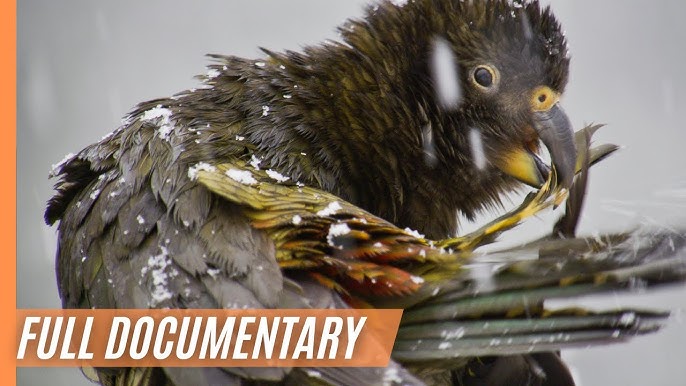This image is a detailed promotional shot for a documentary, featuring a close-up of a bird set against a gray, snowy backdrop. Dominating the left side is a vertical orange border. At the bottom left, an orange text box stretches partway across the image, containing the white text "Full Documentary" or "Fuel Documentary". The bird, the central focus, is captured in a side profile, highlighting its dark brown head and neck accented with yellow around the eye and on the prominent beak. Its feathers display a mix of brown, yellowish, gray, with hints of orange and green. The bird appears to be gripping or interacting with something resembling a stick. This compelling composition draws attention to the bird's intricate details, making it the standout subject against the wintry background.